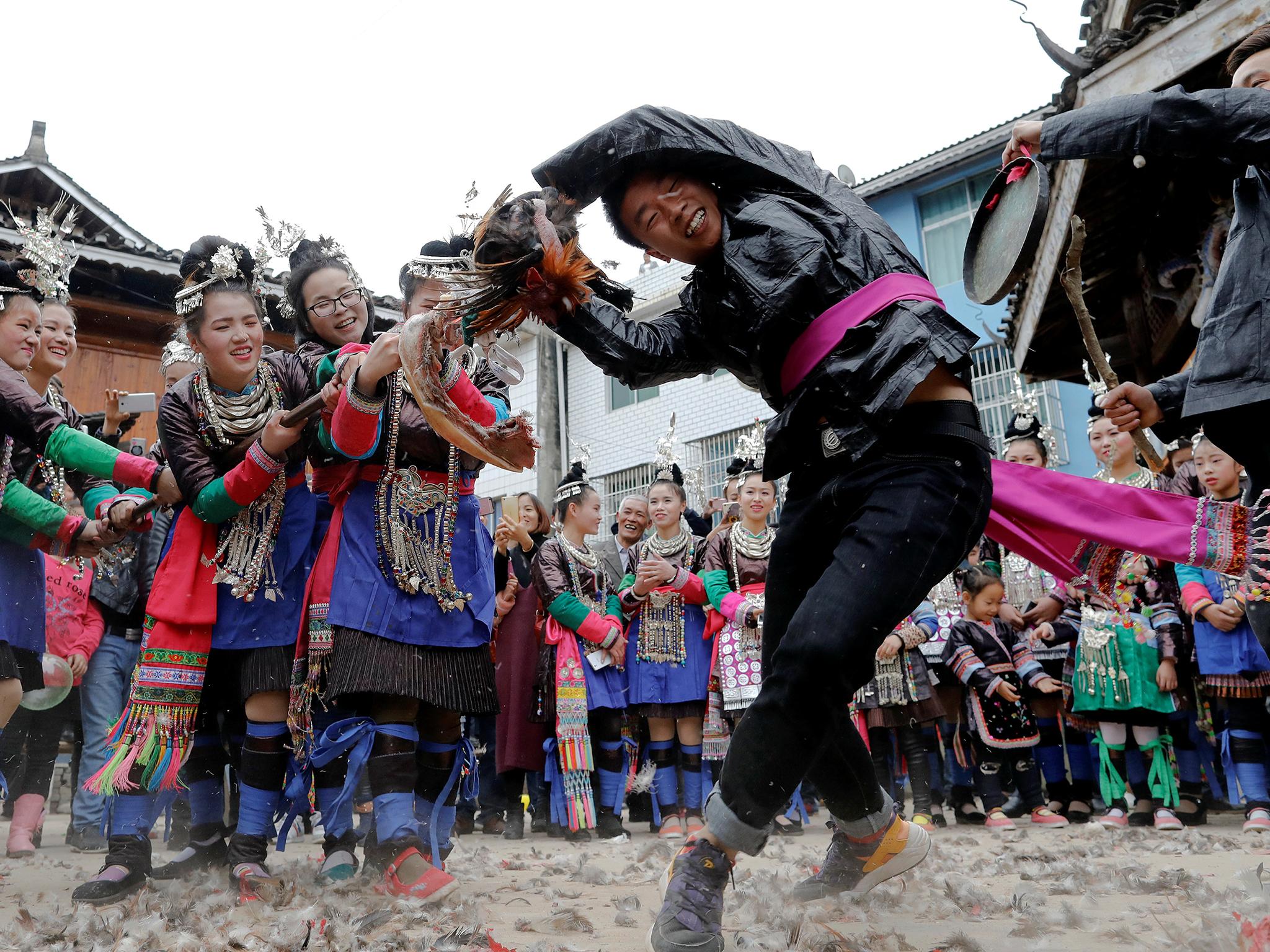In this vibrant photograph, a diverse group of individuals are engaging in what appears to be a celebratory or ceremonial scene, rich in traditional and modern contrasts. At the center is a man distinctly standing out in contemporary clothing, including a black top, cuffed jeans, sneakers, and a pink scarf. He is energetically pulling on a long, large rope or stick, which is gripped by a line of five women to his left. These women are adorned in intricate, colorful traditional attire, featuring blue dresses with green and red accents, accented with numerous silver necklaces, bracelets, and tassels. Their festive clothing, possibly indicative of rural or ceremonial Asian culture, shines brightly with tones of blue, black, and red. 

Surrounding the central figures, more people in similar traditional dress appear to be participating or observing, adding to the lively and communal atmosphere of the event. To the right side of the image stands another man, dressed in non-traditional wear, striking what looks like a gong with a wooden stick, contributing to the musical rhythm of the scene. The background is filled with a crowd of children and adults alike, all donned in festive clothing and tennis shoes, dancing and celebrating on the sandy ground. The overall mood is one of joy, unity, and cultural celebration, with smiles all around and a mix of sounds and colors.